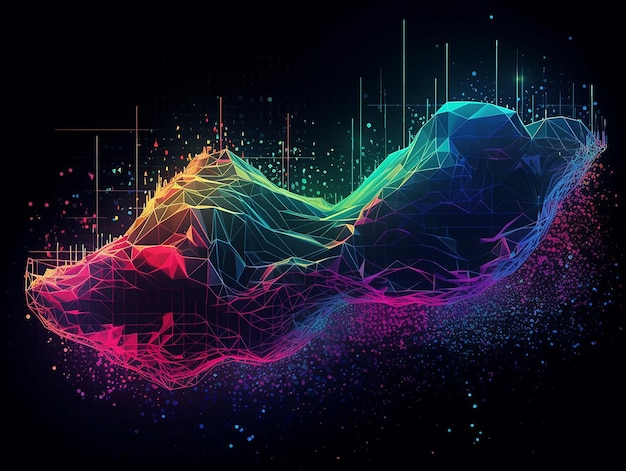This image is a computer-generated graphic featuring a horizontal rectangular composition with a stark black background. At the center, a vibrant, geometrically-shaped 3D object resembling two mountain peaks commands attention. The left peak is pointier but shorter than the right. The object is composed of various interconnected geometric shapes with different elevations, outlined by brightly neon colors spanning the full spectrum of the rainbow—from purple at the bottom to hot pink, transitioning through green, blue, yellow, and orange to red at the top. Additionally, numerous dots and lines, resembling sprays of paint and stars, scatter throughout the image. Vertical lines also emanate from the top of the peaks, extending upward and integrating with the splatters. The intricate interplay of shapes, colors, and lines creates a mesmerizing, otherworldly visual experience against the minimalist dark backdrop.